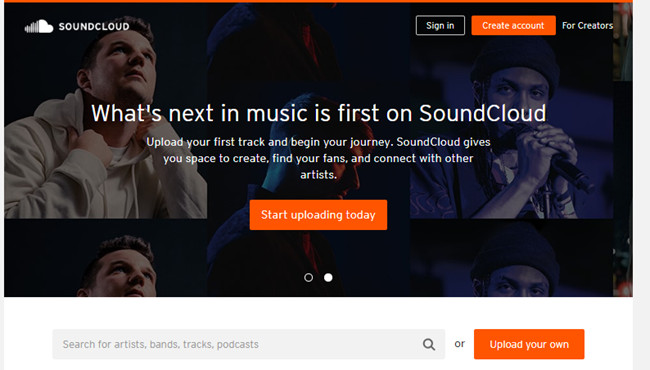The image is a promotional screenshot from the SoundCloud website. The top left corner prominently displays the SoundCloud logo. To the right, there are three interactive tabs: "Sign In," an orange-highlighted "Create Account" button, and "For Creators." Centered in the background is a large image featuring a Caucasian male wearing a white hooded pullover sweatshirt. This image is repeated twice – in the middle and at the end of the sequence – with the final figure appearing to be a darker-skinned male set against a dark background. Positioned centrally in the image, the text reads: "What's next in music is first on SoundCloud. Upload your first track and begin your journey. SoundCloud gives you space to create, find your fans, and connect with other artists. Start uploading today." Below this text, there are two navigation dots indicating the presence of multiple pages. The first dot is empty, and the second dot is filled in white, signifying that the user is currently viewing the first of the two available pages.